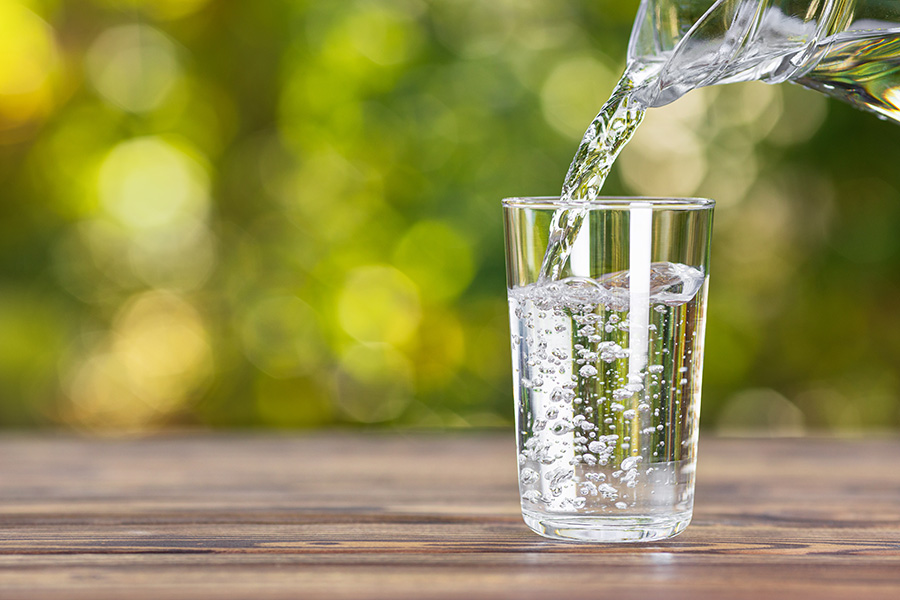The photograph captures a close-up scene of a clear glass pitcher pouring water into a tall cylindrical water glass on a medium brown wooden tabletop. The water, clear and slightly bubbling as it flows into the glass, is about three-fourths full, with a soft splash and bubbles forming at the surface. The background is blurred, showcasing various shades of green, white, and off-white, suggesting an outdoor setting with trees or bushes. Reflections in the glass create a white line, adding to the image's detail and complexity. The tabletop features a brown and tan striped layered wood pattern, complementing the overall composition.